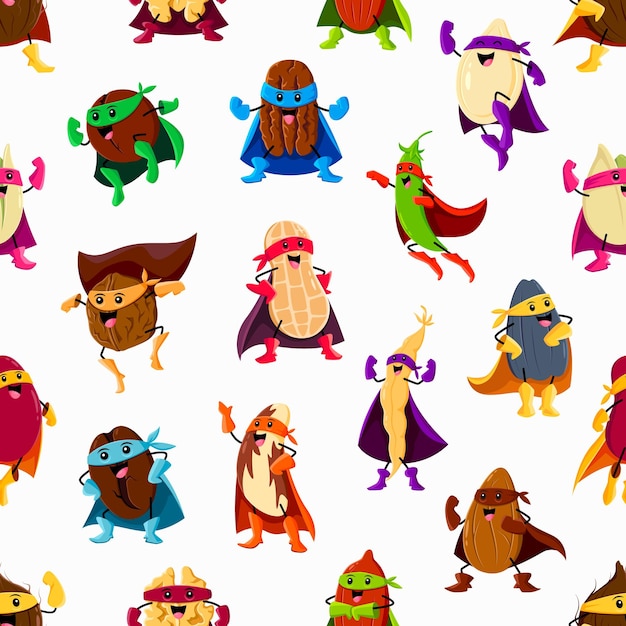The image is a whimsical wallpaper featuring various colorful cartoon characters, primarily depicting different types of food as playful superheroes. Each character is embellished with a distinct cape and mask, with the majority sporting bandanas over their eyes. Among the characters, there's a smiling peanut in a red mask, red boots, red gloves, and a purple cape, exuding a heroic charm. Nearby, a cocoa bean dons a blue mask and cape, while other hero-foods include a walnut, a coconut, a pecan, a jalapeno, an onion, and a gourd. All characters are set against a white background, making the vibrant colors—orange, red, blue, green, and purple—pop distinctly. No text is visible in the image, emphasizing the lively, imaginative designs that could easily be from a children's cartoon.